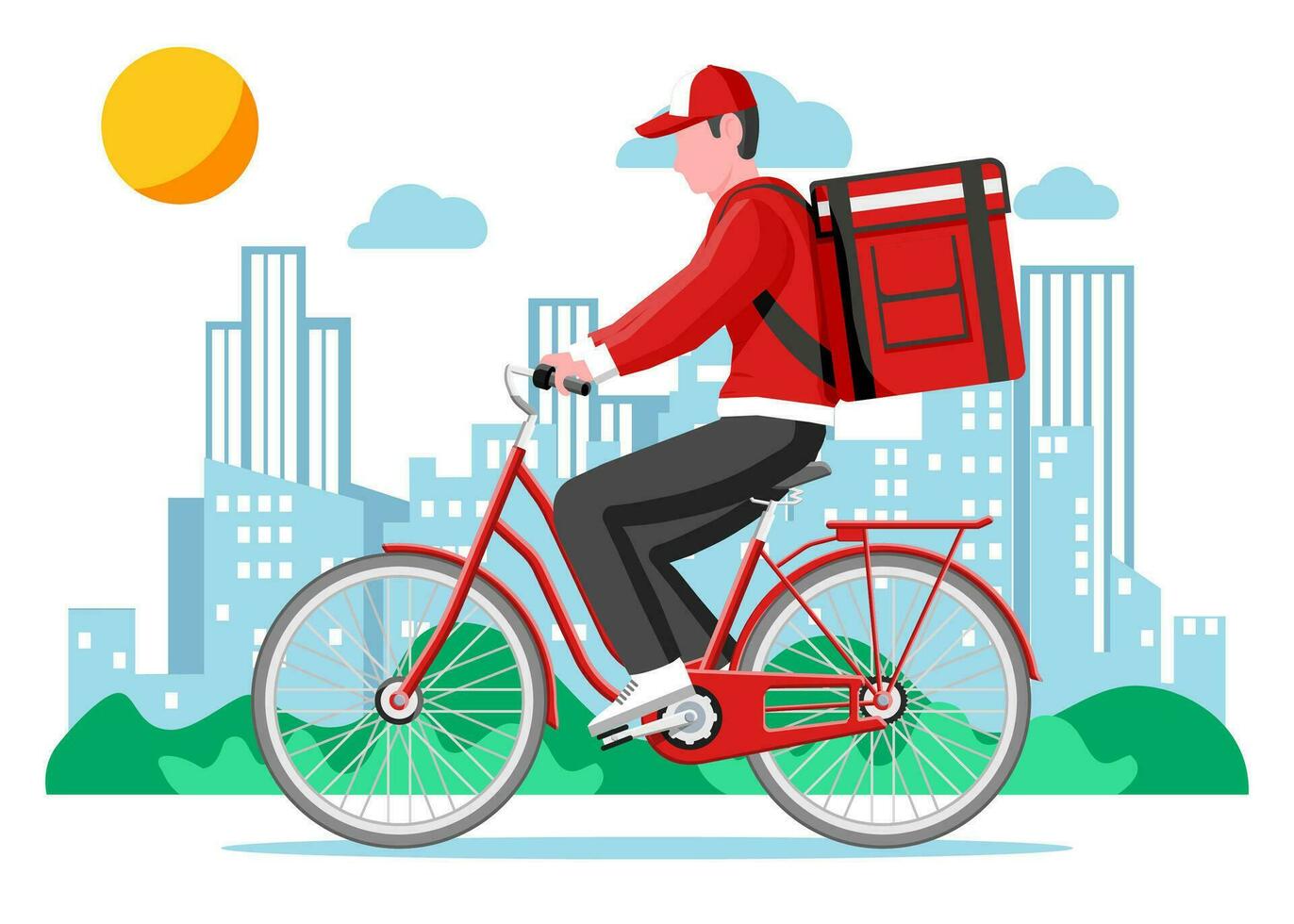The image is a cartoonish depiction of a Caucasian male bike messenger donning a red sweatshirt and a red and white baseball cap. He has short dark hair and is equipped with a big, red square delivery bag on his back. He is dressed in black pants and white shoes, riding a red bicycle with gray tires. The scene is set against a blue city skyline featuring tall buildings with white windows. The sky above is white with three light blue clouds and an orange and yellow sun in the top left corner, displaying a darker hue on the bottom right part. Beneath the cityscape, there are dark green wavy hills with lighter green smaller hills in front. The messenger, seen traveling to the left, is positioned in the foreground with vibrant greenery, including bushes and trees, accentuating the scene.